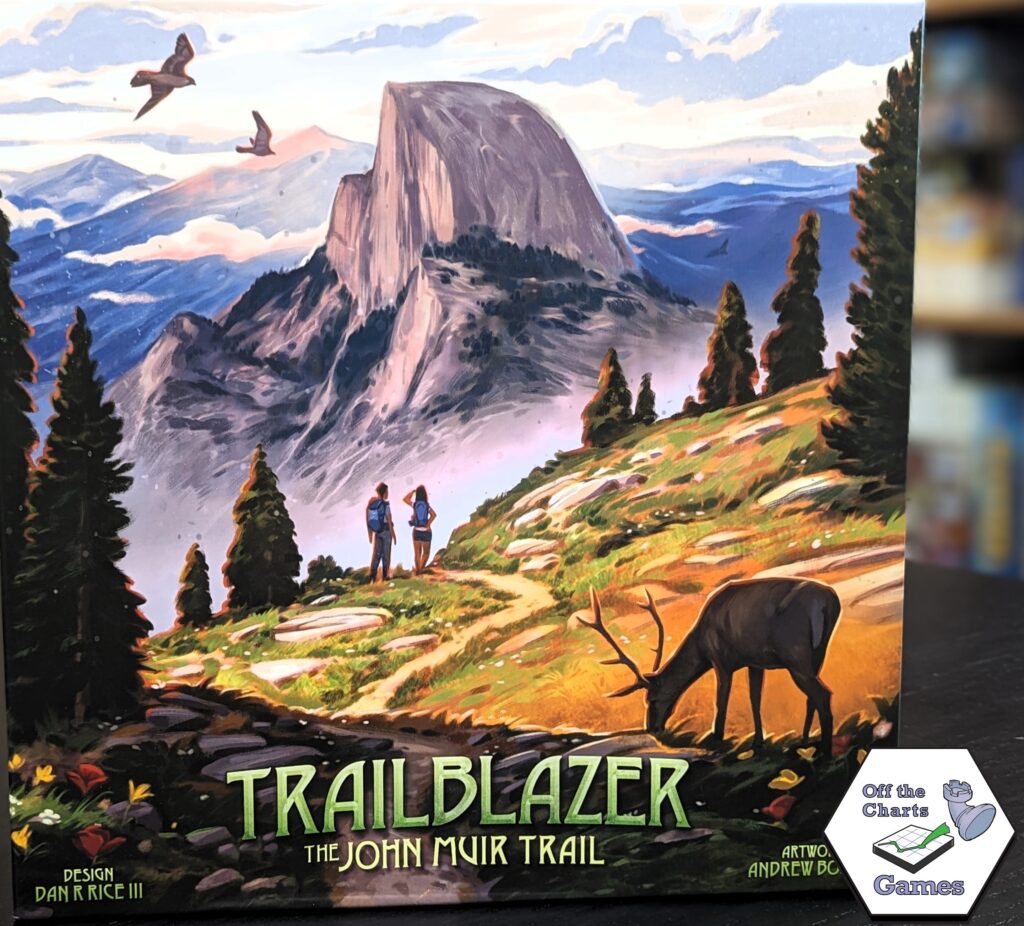The image depicts a vibrant, colorfully illustrated board game cover centered prominently. The title, "Trailblazer: The John Muir Trail," is inscribed in capital letters at the bottom center. To the left, it credits Dan R. Rice III as the designer, while on the right, partially obscured by a white hexagon, it attributes the artwork to Andrew Bo... (last name cut off). The hexagon bears the logo "Off the Charts Games."

The artwork showcases two hikers, a man on the left wearing long pants and a woman on the right in shorts, both equipped with backpacks, walking along a trail towards a towering, rocky mountain in the background. A deer, head down grazing on grass, appears in the bottom right corner of the foreground. The scene is enriched with additional nature details such as flying birds, stones, rocks, trees on the sides, a blue sky, and scattered clouds. A bed of flowers can be spotted near the designer's credit.

The board game box, set on a table, appears in the foreground with a blurred store setting or additional board games visible in the background. The palette includes vivid shades of orange, green, blue, white, gray, red, and yellow, enhancing the overall detailed and immersive scene.